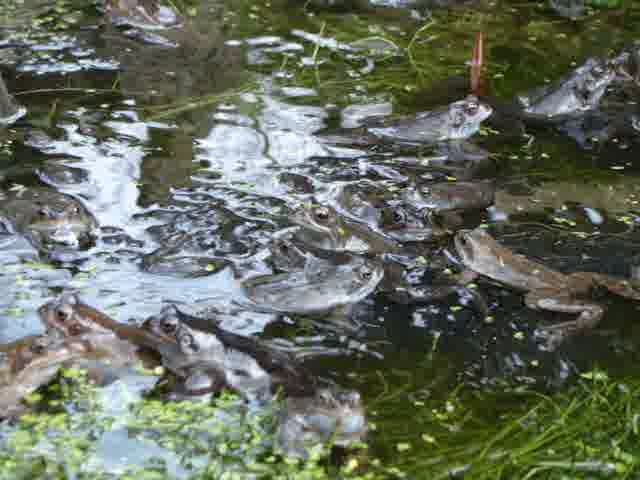The image depicts a small, murky pond teeming with frogs. The water, slightly blurred and filled with various artifacts, displays a dynamic interplay of reflections and the natural environment, making it difficult to distinguish between the frogs and their surroundings. Numerous frogs, almost uniform in size and predominantly gray and brown, are scattered across the scene. Some frogs have their heads perched above the water, while others appear in mid-swim. Pond grass, green leaves, stems, and seaweed-like vegetation are clearly visible, adding layers of texture to the scene. Notably, two frogs are situated in the lower-left corner—one gray and one brown—while another is positioned in the upper mid-right. Rocks and yellow floating debris intersperse the pond, sometimes mimicking the shape of the frogs, adding to the overall visual complexity. One distinct frog on the right seems poised to jump, with its legs ready for action, contributing to the liveliness captured in this tightly-cropped, slightly zoomed-in frame.